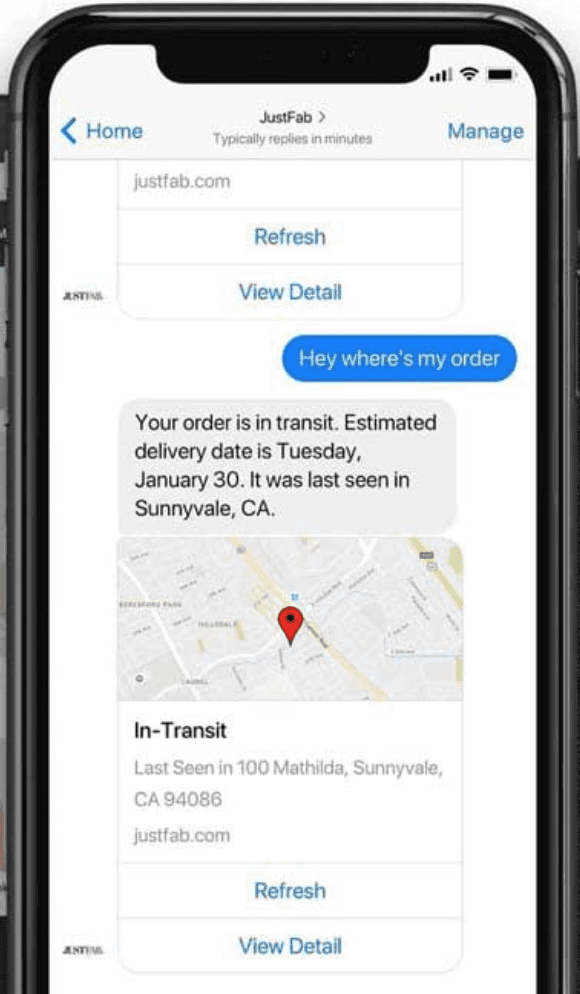A detailed caption for the image could be:

"A screenshot from a phone displaying the JustFab application. The phone has a black border, and the visible part of the screen has a white background. At the top of the screen in blue text, it says 'Home' with an arrow pointing to the left. Centered in black text is 'JustFab,' followed by a smaller font that says 'Typically replies in minutes.' On the right side, also in blue text, it reads 'Management.' Below this header, in gray, it states 'JustFab.com.' Further down, there is a blue hyperlink labeled 'Refresh,' followed by another blue hyperlink 'View Detail.'

A blue oval button on the right side of the screen features white text saying, 'Hey, where's my order?'. Beneath this, there is a gray rectangular section with black text that reads: 'Your order is in transit. Estimated delivery date is Tuesday, January 30. It was last seen in Stanleyville, CA.' Below this message, a map is displayed with a red marker indicating the last known location of the order.

Underneath the map, the text reads 'In transit' in black, followed by 'Last seen in 100 MATHILDA, Sunnyvale, CA 94086' in gray. At the bottom, 'JustFab.com' is mentioned again in gray text. Lastly, there are two blue hyperlinks stating 'Refresh' and 'View Detail,' respectively. The bottom part of the screen is cut off and not visible."

This caption provides a thorough description of the various elements visible in the screenshot.